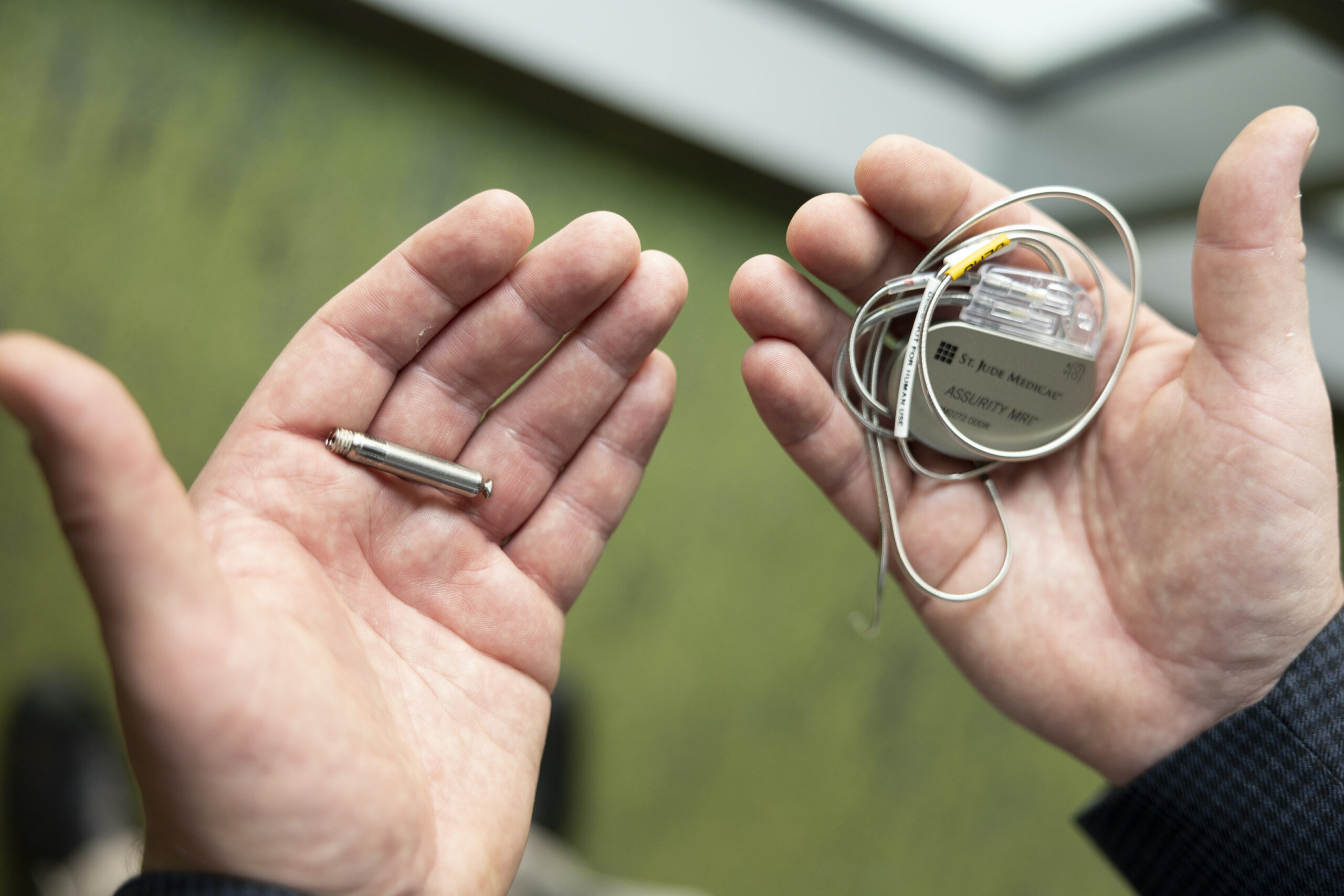The image depicts a pair of human hands, palm-up, set against a backdrop that includes the sleeves of a gray coat jacket with black check patterns. The hands are indoors, beneath a skylight or window. The left hand grasps a small, stainless steel tube, possibly a battery or antenna. The right hand holds a metallic chamber inscribed with "St. Jude Medical Assurity MRI," accompanied by a square logo featuring nine black dots. Surrounding the chamber is a coiled wire terminating in two clear plastic heads. The device appears to be an electronic medical apparatus, likely a pacemaker, indicative of a person's medical journey.